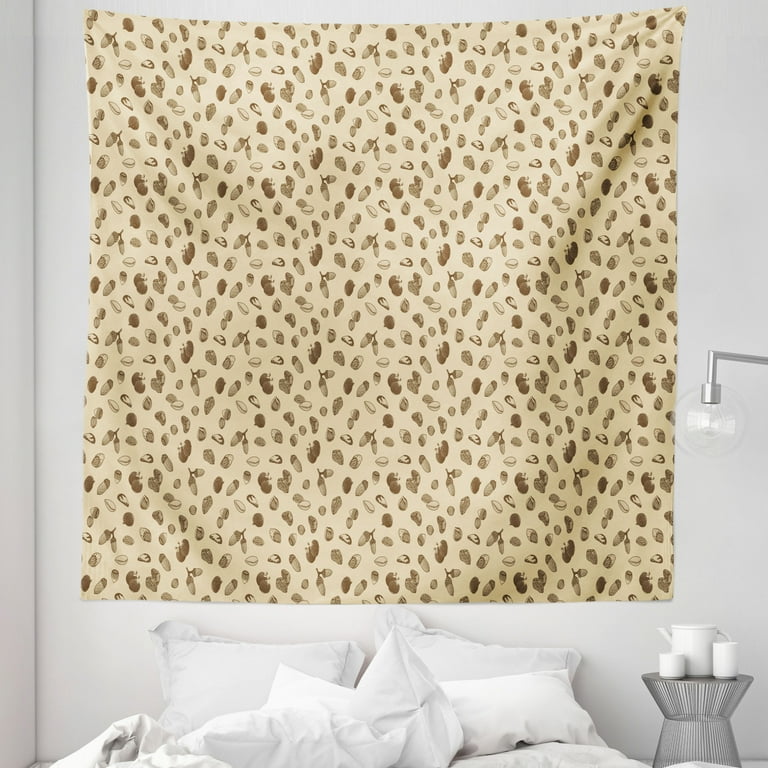The photograph depicts a bedroom with a predominantly white decor. The unmade bed features disheveled white pillows and sheets. To the right of the bed stands a grayish-silver nightstand supporting a white ceramic teapot alongside two cups. Above the bed, a large, light yellow or beige sheet is tacked to the wall, adorned with a detailed pattern of brown and gray acorns—some singular and others in pairs. Extending from the right side of the wall is a silver arm with a white spherical light fixture dangling from it. The background exhibits a light grayish hue, contributing to the room's serene and minimalistic aesthetic.